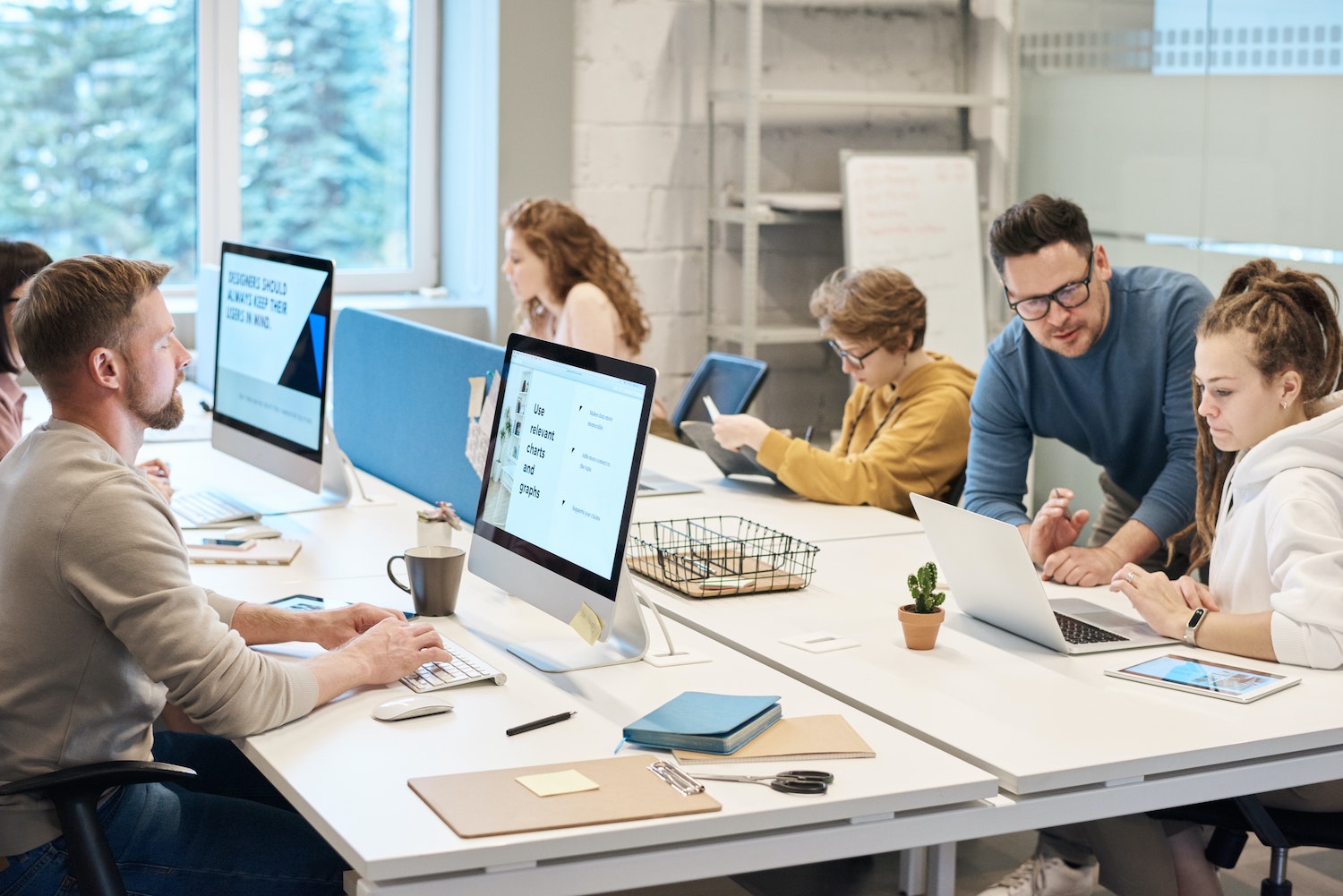In a spacious, contemporary open-office environment with white brick walls and a large window showcasing trees outside, a group of six workers are engaged at a sizable double-sided white table. The table, cluttered with various work objects like laptops, Apple displays, notebooks, folders, scissors, clipboards, pens, and coffee cups, reflects a busy and collaborative atmosphere. On the right side of the image, a young woman with brown dreadlocks in a white hoodie is aided by a bespectacled man in a blue long-sleeve shirt, leaning over her laptop. Next to them, a 20-something woman in a golden hoodie is focused on writing in a notebook. Across from them, two individuals are immersed in their work using Apple Magic Keyboards and Mice, with one screen displaying the message, "Use relevant charts and graphs." The white shelving against the distant wall is conspicuously empty, adding to the staged feel of the office.